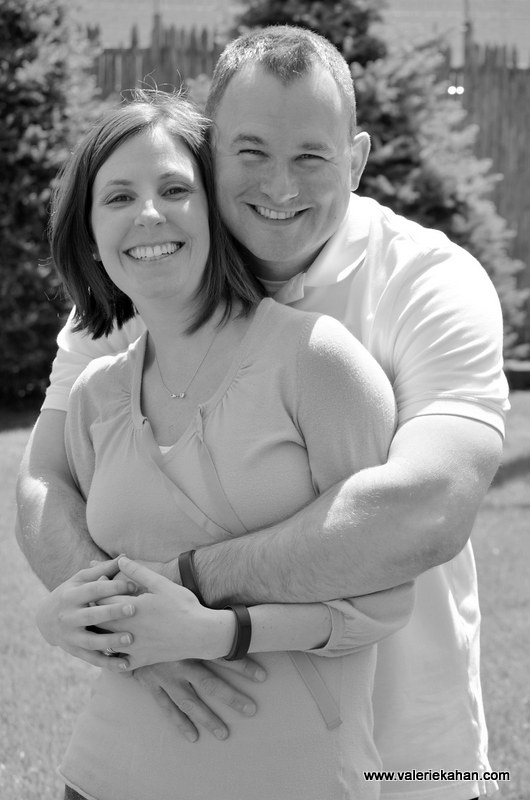This black and white photograph, taken by a professional photographer (www.valeriekahan.com), captures a joyful couple embracing each other outdoors in front of blurred pine trees and a fence. The man, who appears to be in his mid-thirties, has short, well-groomed light-colored hair and is wearing a light polo shirt along with a black bracelet. He stands behind the woman, wrapping his arms around her waist, and they both face the camera with broad, happy smiles. The woman, also appearing to be in her mid-thirties, has shoulder-length brown hair and is dressed in a light, long-sleeve top with a necklace. She clasps her hands over the man's hands, showing that she is wearing a matching black bracelet. The photograph exudes warmth and intimacy, reflecting the couple's close bond.